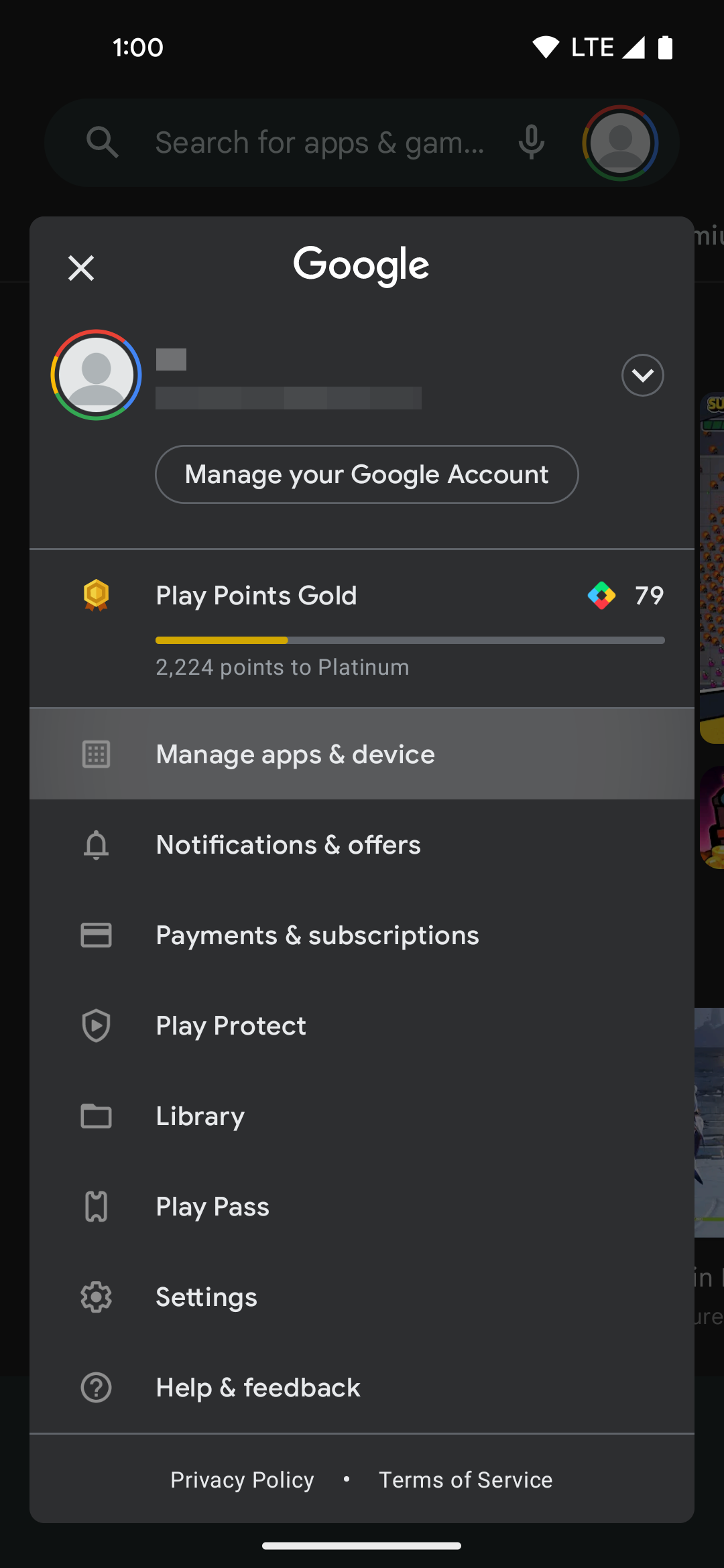The smartphone screenshot showcases a detailed interface of a Google Play Store account. At the top, the time is displayed as "1" in bold white font, suggesting military time, while adjacent icons indicate various statuses: a full WiFi signal, LTE data connectivity, robust signal strength symbolized by a filled triangle, and a fully charged battery.

Beneath this, a search bar appears faded in gray and white with a magnifying glass on the left and partially visible text indicating "search for apps and games." Beside the search bar, an icon resembling a microphone is displayed, flanked by the Google logo—a silhouette of a person encircled by red, blue, green, and yellow on a light gray background.

Prominently in the center, a large black rectangle with a bold white "Google" at the top stands out. An 'X' on the left allows for dismissal of the window. The user's name is obscured for privacy, and below, an oval button labeled "Manage your Google account" in bold white offers account management options.

The Play Points section follows below, featuring a gold and brown hexagonal icon with ribbon details indicating a reward. It reads "Play Points Gold" with a tally of "2,224 points for platinum." To the right, the number "79" appears next to a tilted square in blue, green, yellow, and red quadrants.

A cascading list of options reveals the first item highlighted with a dark gray border, labeled "Manage apps and devices" next to a square with multiple white dots. Subsequent options include "Notifications and offers" marked by a bell icon, "Payments and subscriptions" symbolized by a credit card image, "Play Protect" featuring a shield with a play button, "Library" indicated by a folder, and "Play Pass" depicted as a ticket stub. Finally, "Settings" are represented by a gear icon, and "Help and feedback" by a circle with a question mark.

At the screen's bottom, in gray text, are links to the "Privacy policy" and "Terms of service," separated by a dot, concluding with a white navigation bar positioned at the bottom of the interface.